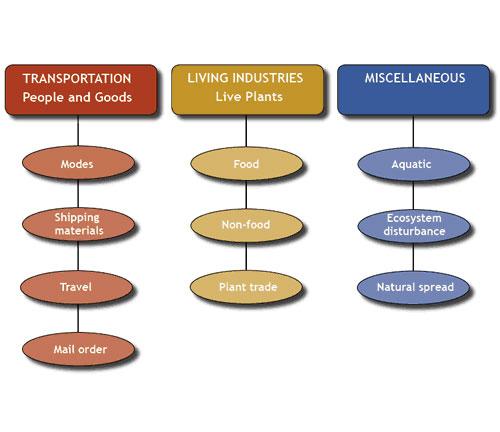In this detailed diagram, there are three vertical columns, each representing different categories and subcategories, with each column having a distinct color scheme for visual differentiation. Starting from the left, the column is shaded in a brownish-red color and has a white-lettered header that reads "Transportation, People, and Goods." This category is subdivided into four sections: "Modes," "Shipping Materials," "Travel," and "Mail Order," each connected by strings to ovals listed vertically down the column.

The middle column, colored in a yellowish-gold hue, is dedicated to "Living Industries, Live Plants." Subcategories branching from this header include "Food," "Non-Food," and "Plant Trade," similarly strung together in a vertical arrangement.

On the far right, the column features a dark blue header labeled "Miscellaneous," with subcategories in a lighter blue tone. These subcategories are "Aquatic," "Ecosystem Disturbance," and "Natural Spread," all aligned vertically with connecting strings and ovals.

Each column's color coding and linked subcategories create an organized chart that visually separates and categorizes information about transportation, living industries, and miscellaneous factors affecting the ecosystem.